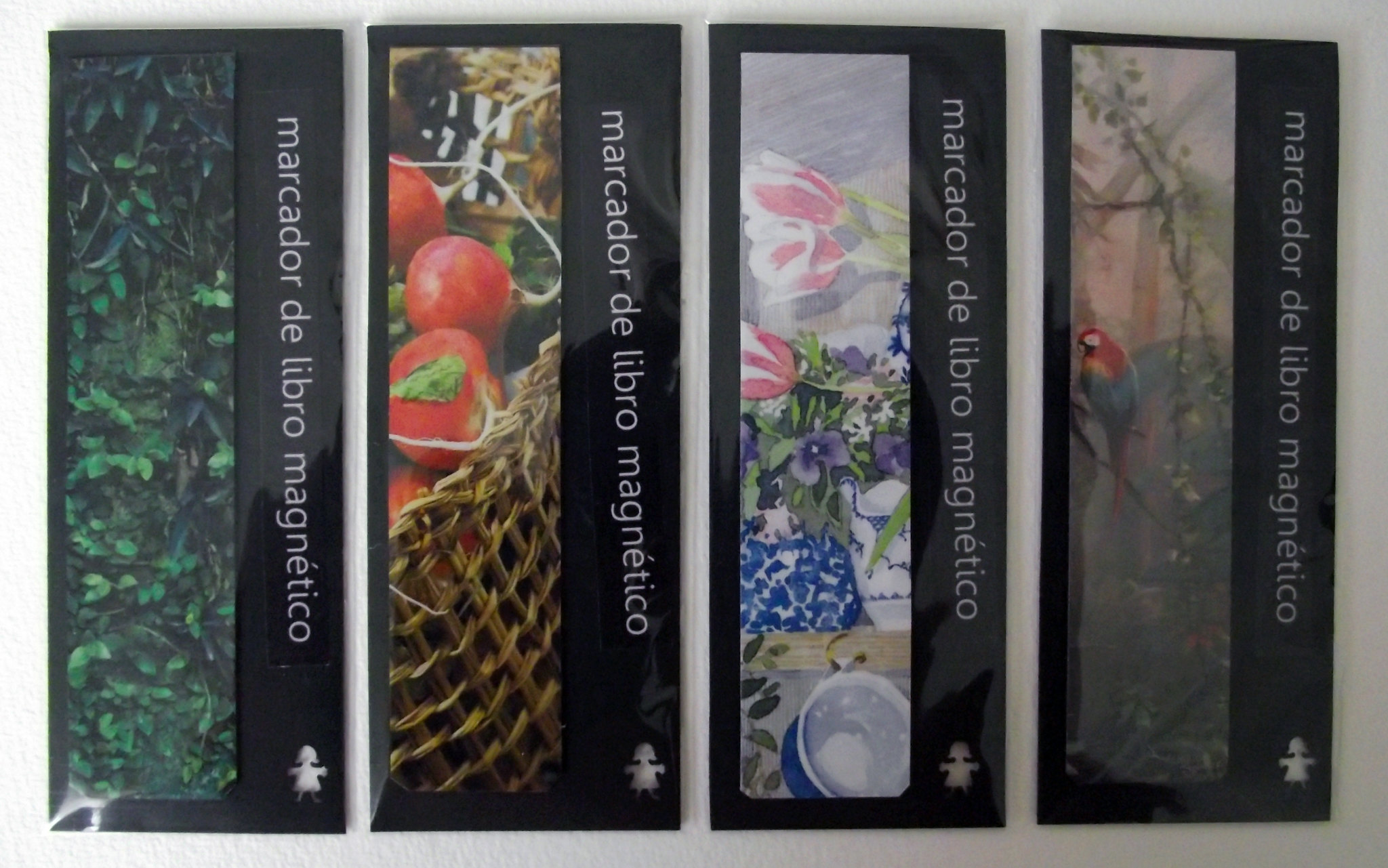The image depicts four rectangular bookmarks, each bordered in black and arranged in a row, filling the entire frame. At the top of each bookmark, the text “Marcador de Libro Magnético” is printed in silver letters against the black background. 

The first bookmark to the left features an illustration of green leaves, reminiscent of those on a vine, that takes up approximately two-thirds of the space. Beside the text, it shows a white outline of a child.

The second bookmark showcases what appear to be green tomatoes with long gray stems, placed in a light brown woven basket.

The third bookmark displays an assortment of flowers in pots. Pink tulips with white accents and green stems, alongside purple flowers that could be lilies, are placed in intricately designed white and blue vases.

The final bookmark depicts a vibrant Amazonian scene with a parrot perched on a branch. The parrot has a striking red head, and its body transitions into a rainbow of colors: yellow, green, blue, and orange. The background features varied greenery, including tall trees resembling dinosaur necks, with some branches and leafy foliage.

Each bookmark also has a small icon of a stick figure of a lady in a dress beneath the text.